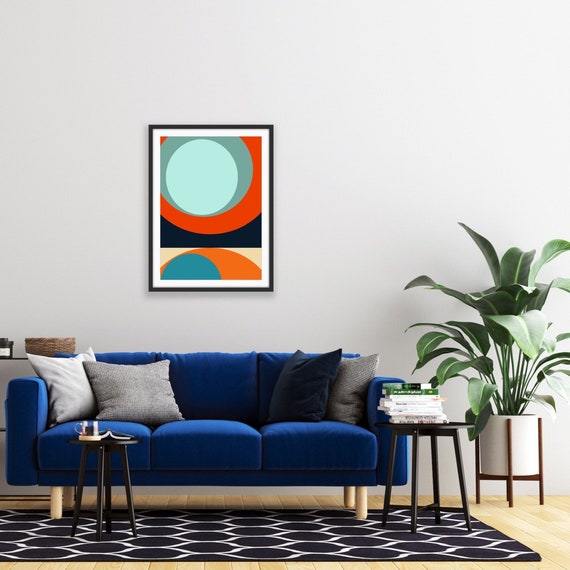The photo captures a stylish living room with a modern aesthetic, perfect for an architectural magazine or a home goods advertisement. The focal point of the room is a blue couch with four wooden stilt legs, adorned with decorative throw pillows in shades of white, gray, and blue. Flanking the couch are two simple black side tables; one is topped with a neat stack of books, while the other holds an open book turned face down and a coffee cup. In front of the couch is a black and white geometric rug that lays over a light beige wooden floor.

The background features a white wall adorned with a modern abstract art piece encased in a simple black frame. The artwork contains an array of colorful orbs and geometric shapes in hues of gray, blue, red, navy, orange, turquoise, and beige, adding a vibrant touch to the room. A tall, green broadleaf plant in a white pot with wooden legs stands proudly beside the couch, contributing a fresh, natural element to the sophisticated decor. Overall, the room exudes a perfectly balanced mix of color, form, and function.